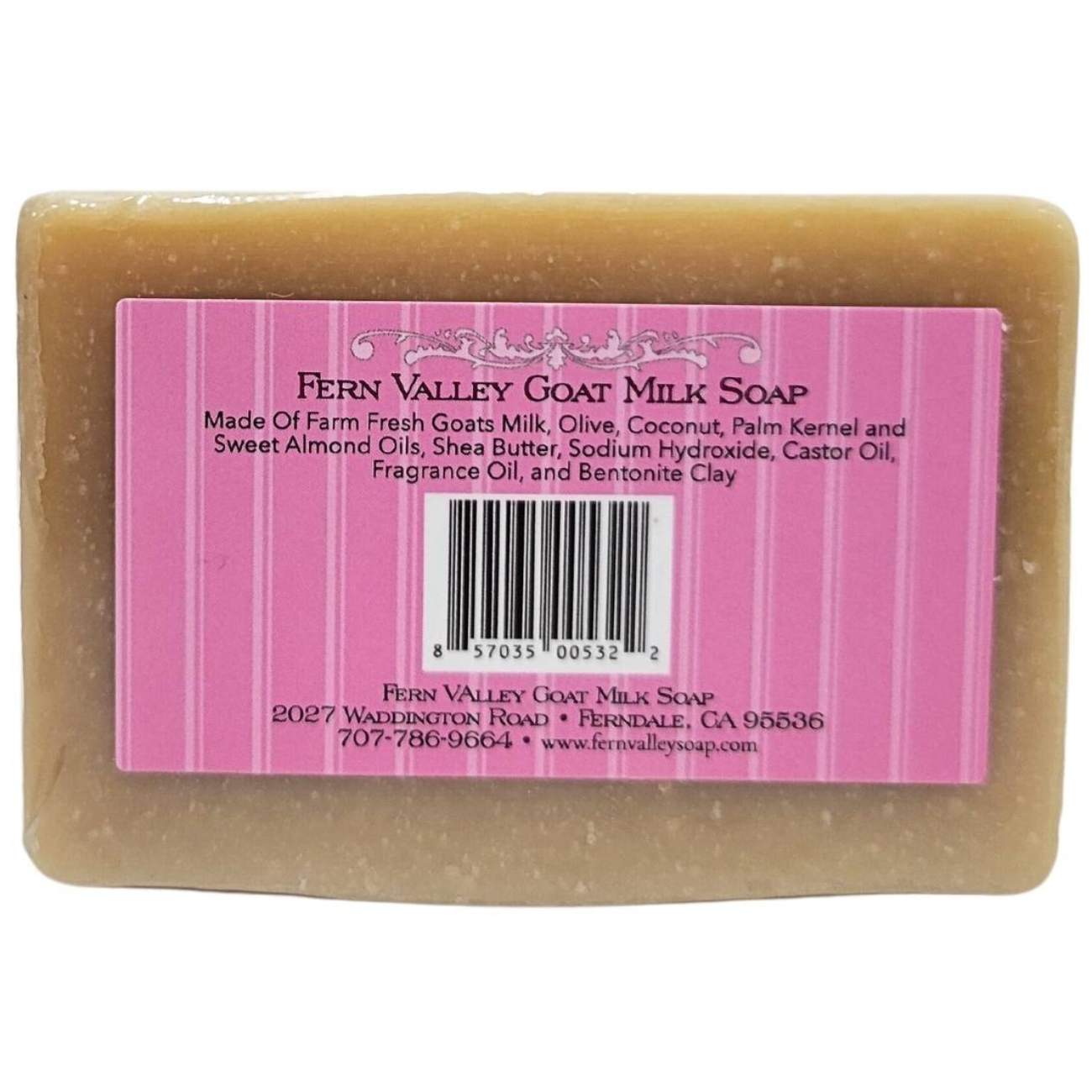The image depicts a rectangular bar of Fern Valley Goat Milk Soap, encased in its plastic packaging. The soap itself is a brownish-yellow color. Prominently displayed on the packaging is a pink label with vertical white lines, covering most of the soap's surface. The label is inscribed with black lettering, which lists the ingredients: farm fresh goat's milk, olive, coconut, palm kernel, and sweet almond oils, shea butter, sodium hydroxide, castor oil, fragrance oil, and bentonite clay. Centrally placed on the label is a barcode with the numbers 8-5-7-0-3-5-0-0-5-3-2-2. Below this barcode, the label provides additional details, including the manufacturer's address: Fern Valley Goat Milk Soap, 2027 Waddington Road, Ferndale, CA, 95536, and contact information: phone number 707-786-9664, as well as the website www.fernvalleysoap.com.